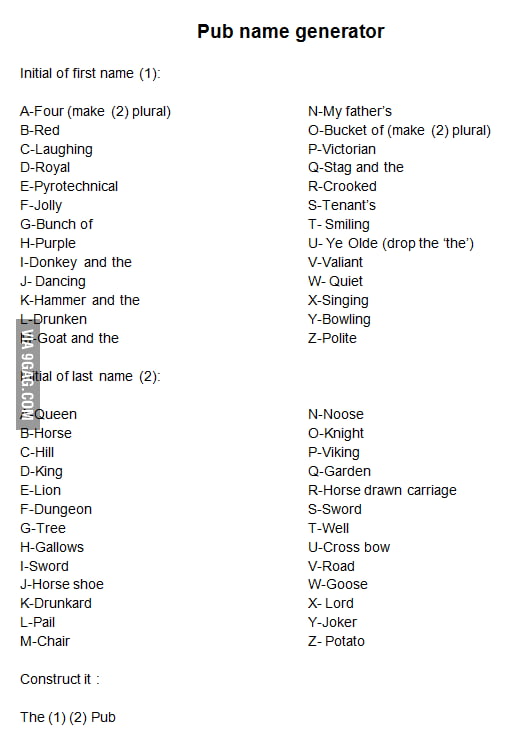The image is a detailed screenshot of a whimsical "Pug Name Generator" tool. At the top of the generator, the title "Pug Name Generator" is prominently displayed. The left side of the image provides options for the "Initial First Name," listing names corresponding to the letters A through L, though only a subset is visible:

- A: Four
- B: Red
- C: Laughing
- D: Royal
- E: Pyrotechnical
- F: Jolly
- G: Bunch of Purple
- H: Donkey and the Dancing
- I: Hammer and the Drunken
- J: Goat and the

Following this, the "Initial Last Name" section lists options for letters A through M:

- A: Queen
- B: Horse
- C: Hill
- D: Long
- E: Lion
- F: Dungeon
- G: Tree
- H: Gallow
- I: Sword
- J: Horseshoe
- K: Drunken
- L: Pail
- M: Chair

Further to the right, the generator continues with options for the "Initial First Name" for letters N through Z:

- N: Constructed
- O: One
- P: Two
- Q: Pug
- R: My Father's
- S: Bucket of
- T: Victorian
- U: Stag and the Crooked
- V: Tenant
- W: Smiling
- X: Yield
- Y: Valiant
- Z: Quiet

The corresponding "Initial Last Name" for N through Z includes:

- N: Singing
- O: Bowling
- P: Polite
- Q: Noose
- R: Night
- S: Viking
- T: Garden
- U: Horse-Drawn Carriage
- V: Sword
- W: Crossbow
- X: Road
- Y: Goose
- Z: Lord

Additionally, under the "Initial First Name" section N-Z and "Initial Last Name" section N-Z, there are other whimsical options:

- Constructed
- One
- Two
- Pug
- Noose
- Night
- Viking
- Garden
- Horse-Drawn Carriage
- Sword
- Crossbow
- Road
- Goose
- Lord
- Jugger
- Potato

At the bottom left of the image is a watermark or bar that says "Via9Gag.com" in white text.

This screenshot captures an amusing and creative tool for generating quirky pug names based on the initials of the user's name.